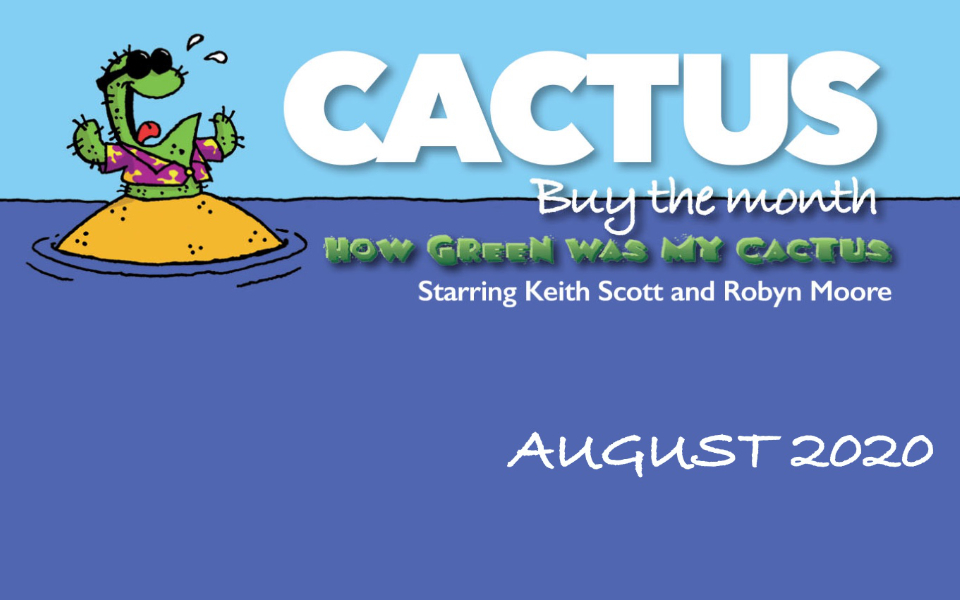The advertisement features a vibrant, hand-drawn or digitally illustrated scene that immediately captures the viewer's attention. The setting is a small sandy island nestled in the middle of a dark blue ocean, with ripples of water highlighted in a deep purple hue. The island itself is a warm beige-orange with scattered black pebbles.

Standing center stage on this tiny island is an animated green cactus character brimming with personality. The cactus dons stylish sunglasses and sports a lively purple Hawaiian shirt adorned with yellow splotches. Its expressive face shows an open mouth with a visible red tongue, giving it a playful and animated demeanor.

Towering above this whimsical cactus, in bold white text, is the title "Cactus by the Month." The words "by the month" are scripted in a smaller, cursive font. Directly underneath in a vivid green, either 2D or 3D font, reads, "How Green Was My Cactus." This is followed by the names of the starring actors, "Keith Scott and Robin Moore," also in white. Finally, at the bottom of the image in italicized, capitalized letters, the text "August 2020" is displayed, indicating the release date of this delightful, likely short film. The background is split between a vast blue sky and the expansive ocean, enhancing the isolated yet charming atmosphere of the scene.